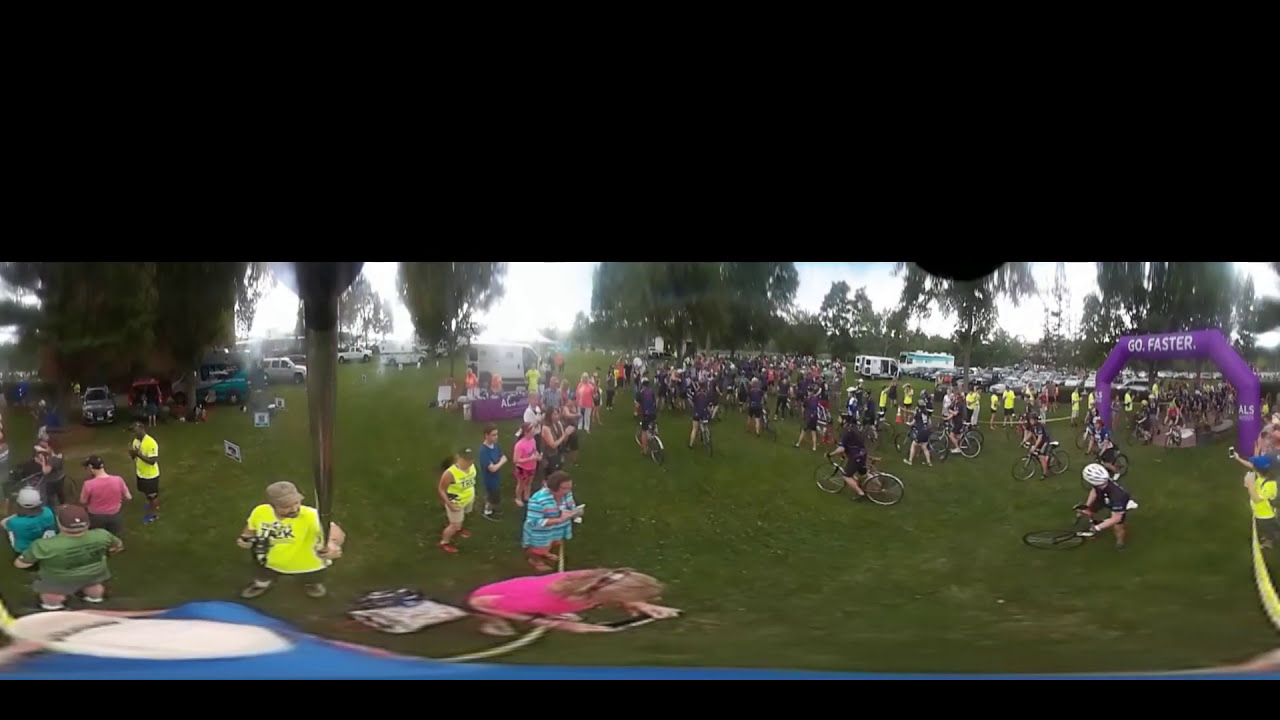The image captures a lively scene at a bike race event, with a wide panoramic view marked by a black border at the top. The background features large, spaced-out green trees with various vehicles, including campers, parked in front of them. Stretching across the grassy field, cyclists and participants, many dressed in purple or darker shirts as well as some in lime green or yellow shirts, are either walking with or riding their bicycles. On the right-hand side, a prominent purple inflatable archway emblazoned with "Go Faster" and an ALS logo stands out as people funnel through it. On the left side, multiple placards are stuck in the lawn, and several spectators are gathered, watching the cyclists intently while some cars are parked under the shade of the trees.